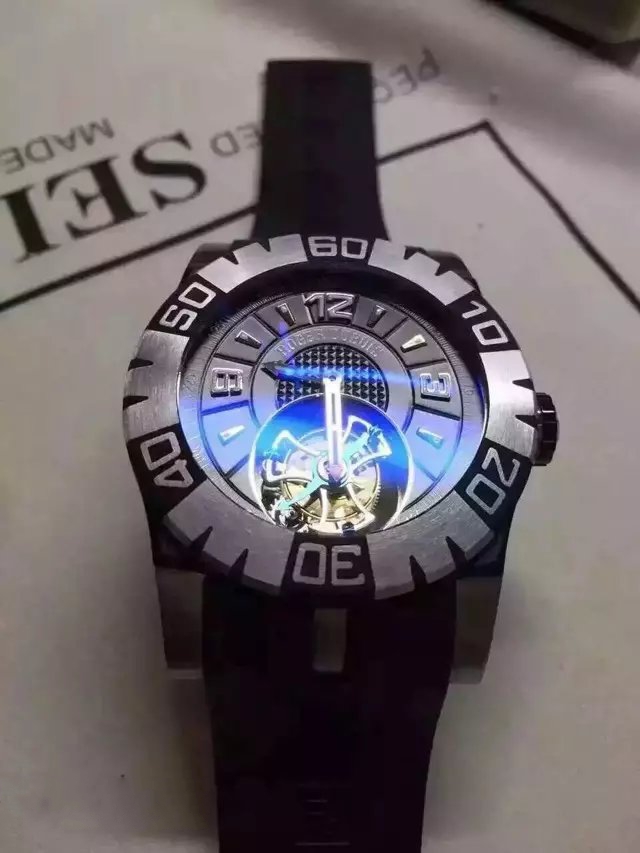A close-up photograph showcases a stylish wristwatch positioned on a piece of paper. The paper is white with a prominent black box, within which the watch is neatly placed. Toward the top left of the frame, text is visible but partially obscured by the watch, rendering it upside down and incomplete. The visible portions of text read "P E," with the watch band concealing the rest, followed by "E D" and, in larger letters, "S E I." Beneath this text, the word "made" appears faintly. 

The watch itself features a sleek black band and a striking silver face, characterized by its metallic sheen and raised numerals. Central to the watch's design is an intricate mechanical component in a subtly desaturated gold tone, comprising numerous small hands and dials that add to its sophisticated aesthetic. The watch's intricate details and craftsmanship dominate the image, resonating with a sense of luxury and precision.